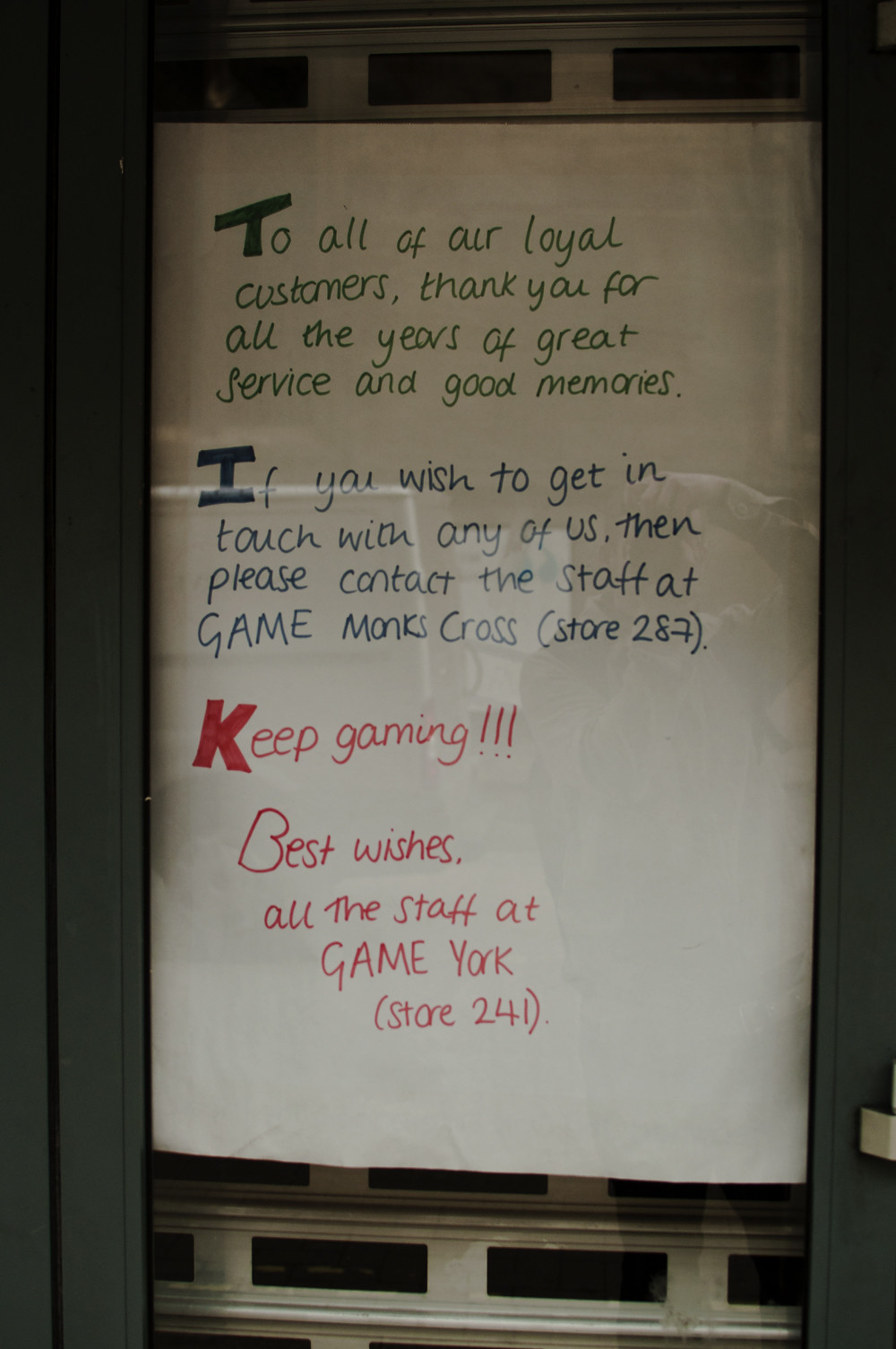In the center of the image, there's a handmade sign prominently displayed on a dry erase board. The board dominates the scene, with an unclear and indistinct background that could suggest it's either indoors or possibly positioned in a store window. The sign features a heartfelt message from a gaming store, written in multiple colors: green, blue, and red letters stand out against the white background. The message reads, "To all of our loyal customers, thank you for all the years of great service and good memories." It continues in blue, "If you wish to get in touch with any of us, then please contact the staff at Game Monks Cross (Store 287)." The closing remarks in red read, "Keep gaming!!!" followed by, "Best wishes, all the staff at Game York (Store 241)." The first letters of "To," "If," and "Keep" are notably bold and enlarged, adding emphasis to the heartfelt farewell. The sign likely signifies the closure of the Game York store, expressing gratitude to its customers and providing contact information for continued support. The setting appears somewhat industrial, hinting that the sign might be placed in a storefront that has ceased operations.